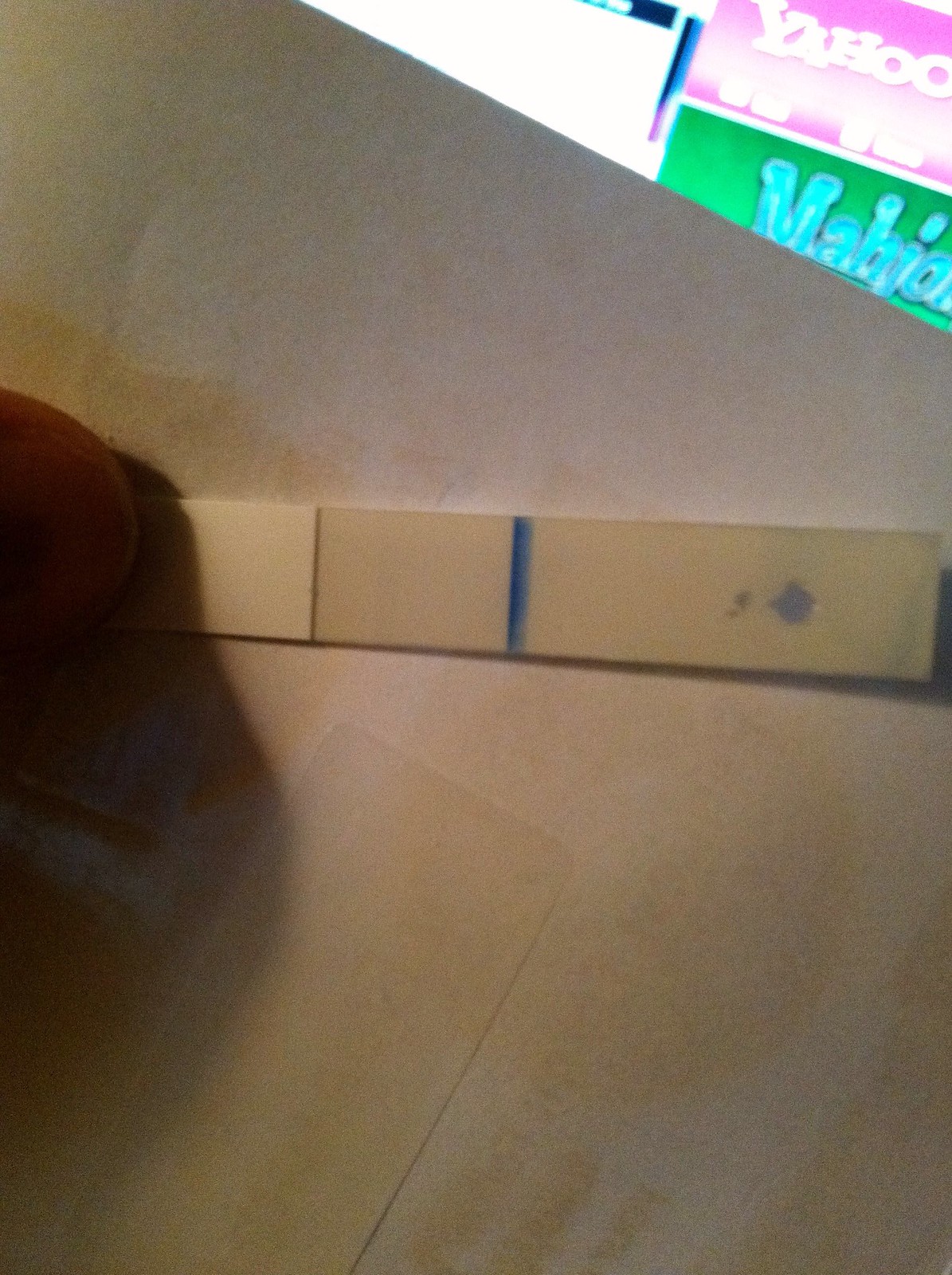In this image, we see a close-up of a pH strip tester, notable for a few distinct blots of greenish-blue liquid. The strip features a solid horizontal line, indicating some sort of measurement. The strip is held by the corner of someone's finger, revealing that it’s still wet from recent use. The background showcases a high-contrast display, where the iconic Yahoo logo is visible. This display might be a television or a computer monitor, though the image is too high-contrast to verify this. Below the Yahoo logo, there's another sign that is not legible due to poor visibility. Additionally, the pH strip or paper appears to have a taped sticker on it and is marked with wet stains, contributing to its dainty yet used appearance.